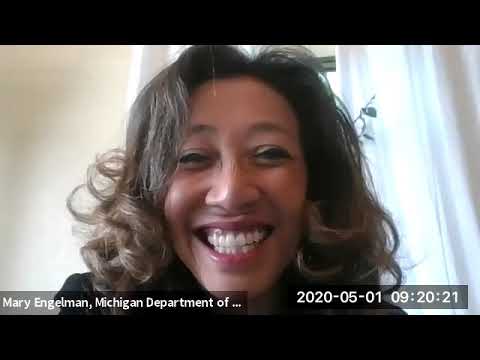The image depicts a close-up, horizontal rectangle photograph of a beaming woman named Mary Engelman. Mary is smiling broadly, showcasing her teeth, with short, wavy, and curly brown hair cascading around her face. Her complexion is slightly dark, and she's wearing makeup that emphasizes her cheerful expression. The photograph is set indoors, likely in her home, as suggested by the white wall and window with white drapes situated behind her, with bright light reflecting on it. Her name and affiliation, "Mary Engelman, Michigan Department of..." is displayed at the bottom of the picture. Below her name, there is a timestamp that reads "2020-05-01, 09:20:21." The overall palette of the image includes shades of white, brown, beige, light blue, red, tan, and gray.